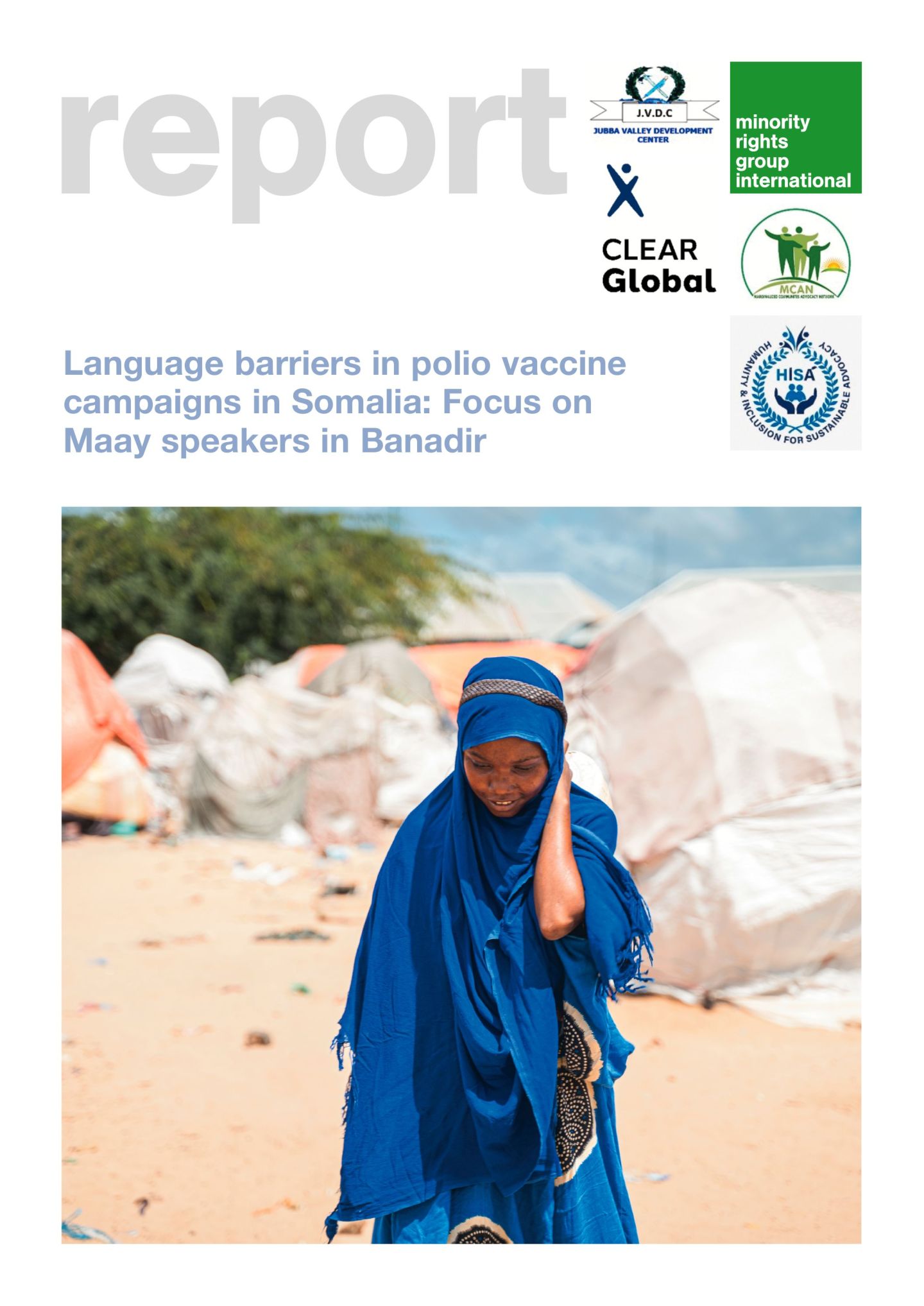The image is a detailed report cover highlighting "Language Barriers in Polio Vaccine Campaigns in Somalia: Focus on Maay Speakers in Banadir." Prominently displayed at the top are the words "Report," with a subtitle beneath mentioning the focus on language barriers. The top right corner features multiple logos, including the Jamba Valley Development Center (a ribbon-like emblem with "JVDC" in the center and a blue X over a black circle), Minority Rights Group International (a green square with the organization's name inside), CLEAR Global, and MCAN (depicted with three figures staring at a sunset). Additionally, the Humanity Inclusion for Sustainable Advocacy logo shows a blue wreath with hands lifting two figures and the acronym "HISA."

Below these logos is an image of a woman clad in a beautifully patterned blue hijab, holding it down with one hand. She stands amidst a sandy, blurred background with white and orange tent-like structures, possibly dwellings, signifying a setting in Somalia. Further elements include blue sky patches, some clouds, and trees in the distance, suggesting a daytime scene. The woman, seemingly deep in thought, is walking toward the camera, emphasizing the human element of the report's focus.